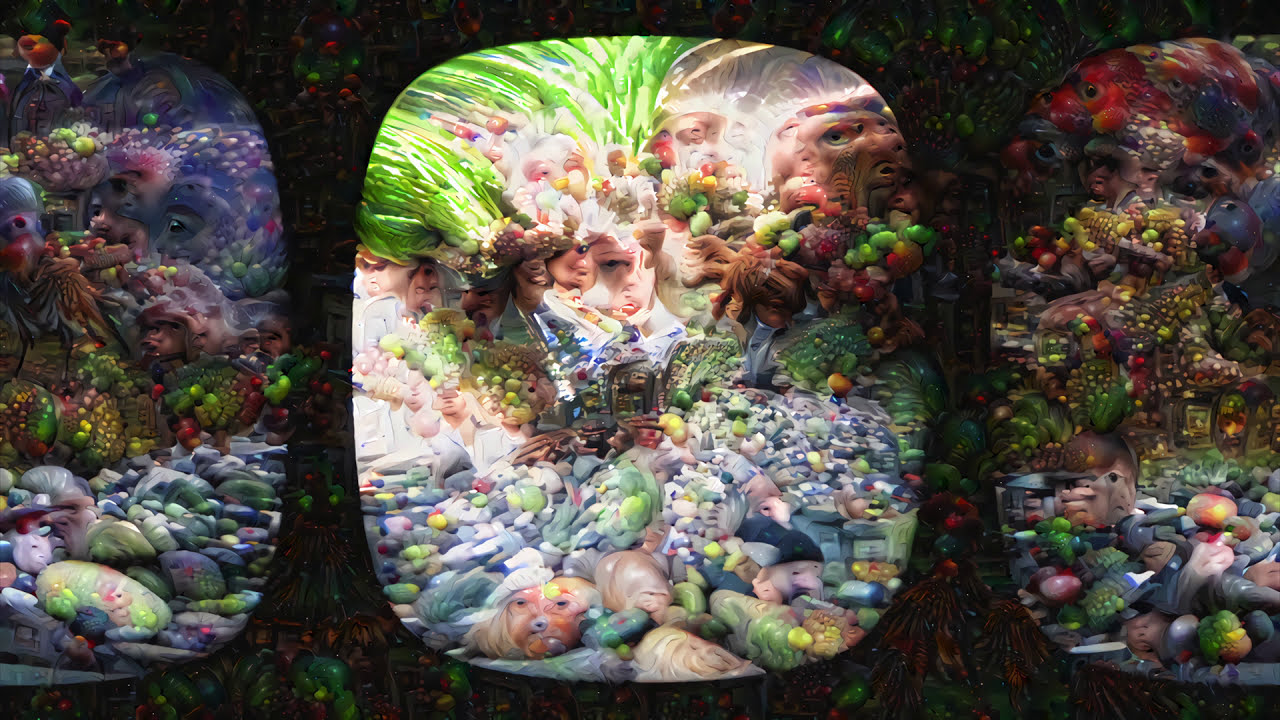The image is a vibrant and surreal collage, reminiscent of a trippy cartoon or comic book strip, divided into three distinct sections. The central section features a square with curved corners and contains a variety of colorful objects including gray and blue koi fish, and various fruits such as lemons, limes, apples, oranges, and peaches. There are also green leafy pieces that might be grass, cabbage, lettuce, or onion tops scattered throughout.

Surrounding this square are multiple, distorted human faces and creatures, with one particularly notable distorted face at the center, bent in a way that draws attention. The background varies in colors from dark green to light green, red, purple, brown, and tan, giving the impression that the wall itself is made of fruit and other organic materials.

In each of the three sections, there's a chaotic assembly of shapes that resemble eyes and faces, each section appearing alive in its own unique way. The objects and characters within these sections are of all imaginable colors—yellow, green, blue, brown, gray, orange, purple, pink—creating a mesmerizing and psychedelic effect. There's no text within the image, and the backdrop, mostly black, intensifies the multitude of colors, making the entire scene appear like an otherworldly, animated dreamscape inside an indoor setting.